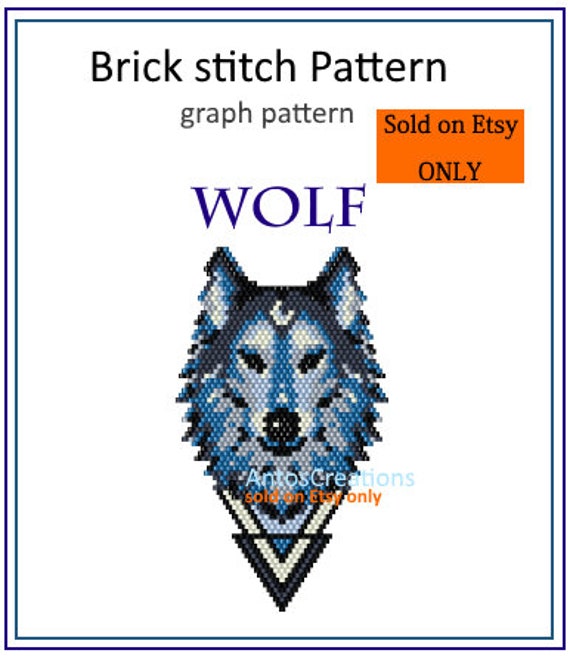The image depicts a detailed cross-stitch pattern advertisement for Anto's Creation, exclusively sold on Etsy. This brick stitch pattern showcases a striking wolf head, predominantly in shades of blue and gray, outlined in black. The wolf, facing directly forward with an intense gaze, has intricate blue highlights and a crescent moon symbol on its forehead. Beneath the wolf's head, on its chest, are two symmetrical triangular patterns combining white, blue, black, and solid charcoal gray. The advertisement features clear black lettering stating "brick stitch pattern" and "graph pattern," with the word "wolf" highlighted in blue. The overall design is bordered by a frame in purple and a type of green. Additionally, an orange sticker at the top right corner emphasizes that this product is "Sold on Etsy only."